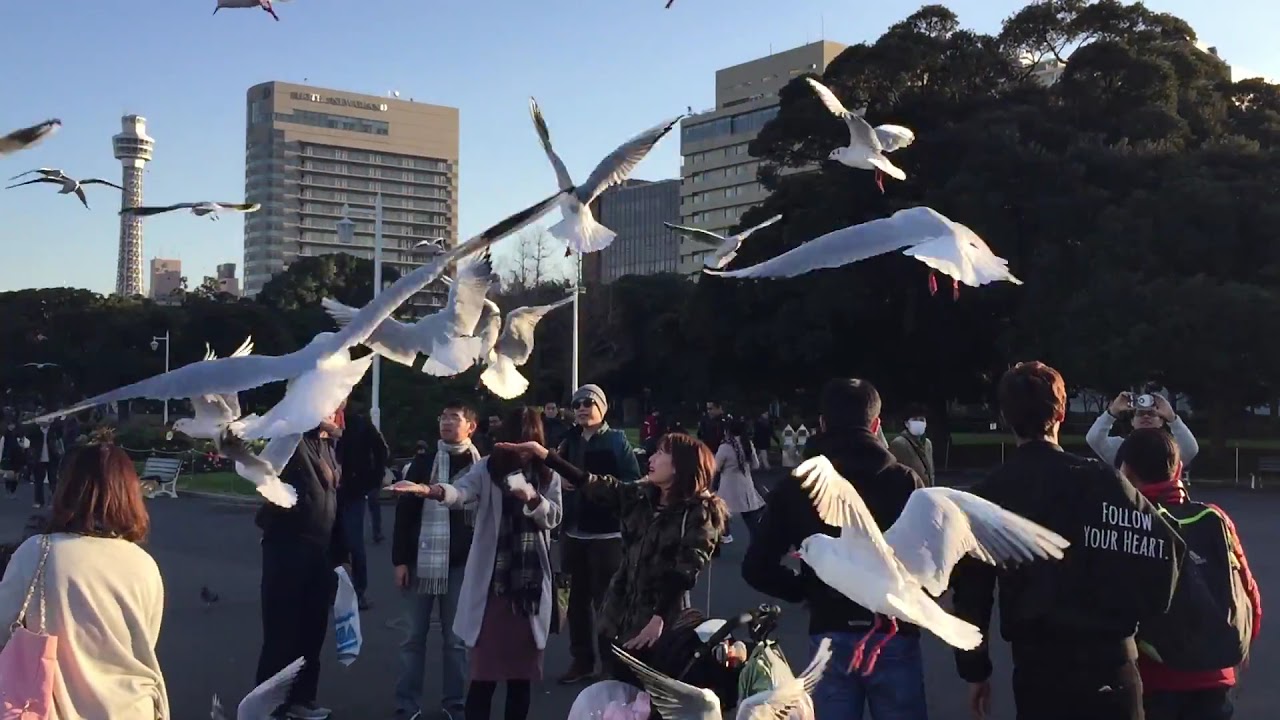The image captures an outdoor scene on a cold day, likely in autumn, depicting a bustling public square where a crowd of warmly dressed people eagerly interact with a lively flock of white seagulls with orange-red feet. The air is filled with the seagulls' frenetic flight, predominantly concentrated in the center of the frame. On the bottom left, a woman with brownish-red hair, wearing a white shirt and carrying a pink purse, stands out. Nearby, there's a stroller laden with bags. The square itself is paved with asphalt, contrasting with the greenery in the background, including several tall, thick trees, some bare of leaves. In the distant background, a mix of high-rise buildings, including a distinctive round tower on the left, create an urban skyline. Among the crowd, a woman can be seen raising her camera to capture the scene of the birds overhead.